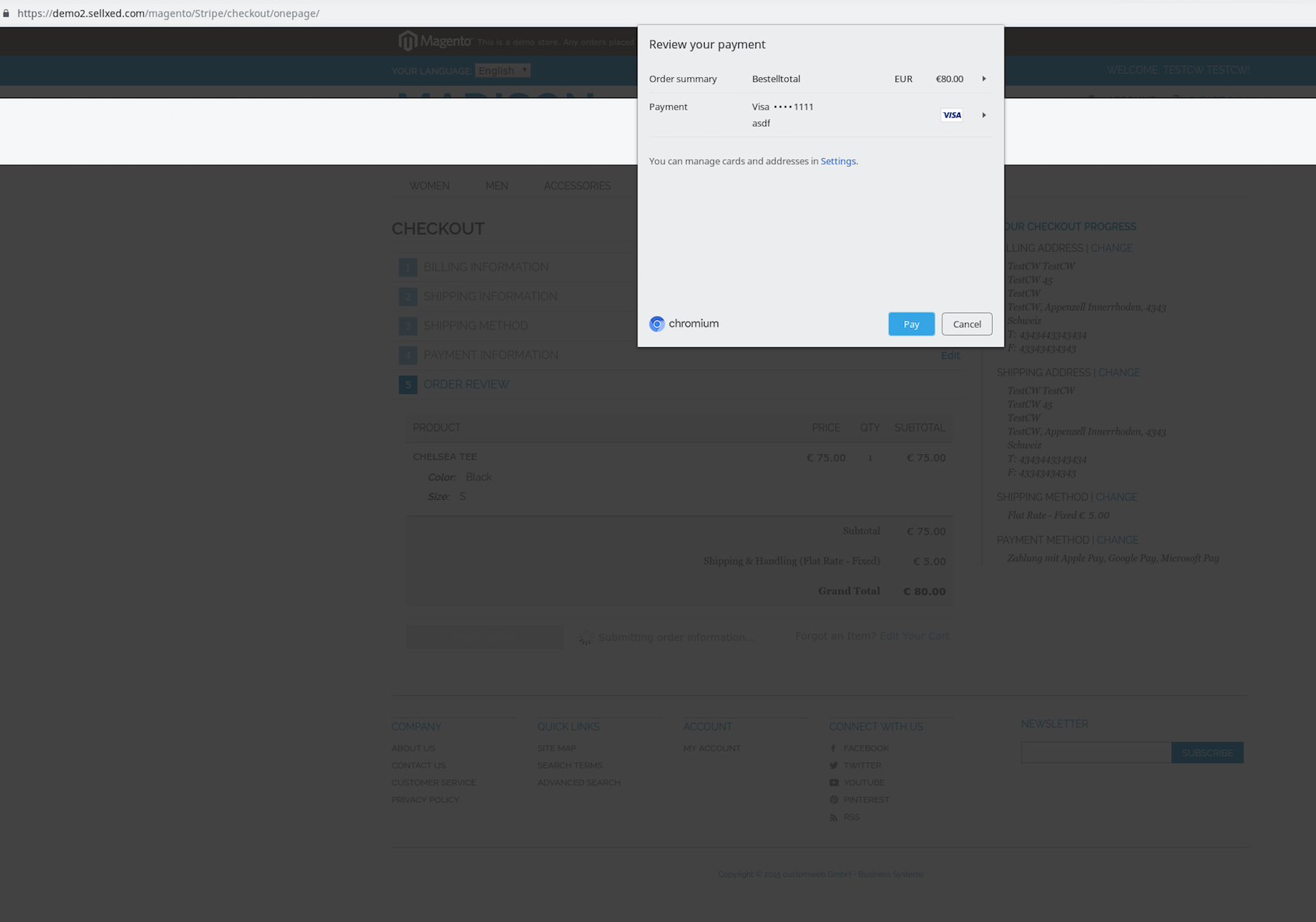This image captures a screenshot of a website featuring a minimalistic design dominated by a white background accented with pale grey details. Currently, the main content is partially obscured by a dark grey opaque overlay due to an active pop-up box. 

At the very top of the screen, a thin bar can be seen, displaying the website address in a diminutive font. The beginning of the URL reads "HTTPS://" but the rest is indistinguishable. Directly below is a darker grey bar, likely an advertising banner, which spans the full width of the screen. Following this is a white navigation bar of similar thickness.

Beneath these elements, partially visible through the dark overlay, is the word "CHECKOUT" on a white background, accompanied by five informational blocks arranged horizontally. Further down, a thin grey strip appears, potentially indicating an itemized total for a sale.

The right side of the screen features a column for additional details, breaking the monotony of the central layout. At the screen's base, there are four main columns containing navigational links, with one column probably dedicated to home information. In the bottom right corner, a site search option is visible.

The prominently displayed pop-up box urges users to "Review your payment." Listed within the box are the user's current payment options, easily changeable if needed. At the pop-up’s bottom right, a blue button labeled "Pay" and a white button labeled "Cancel" offer final steps for the user.